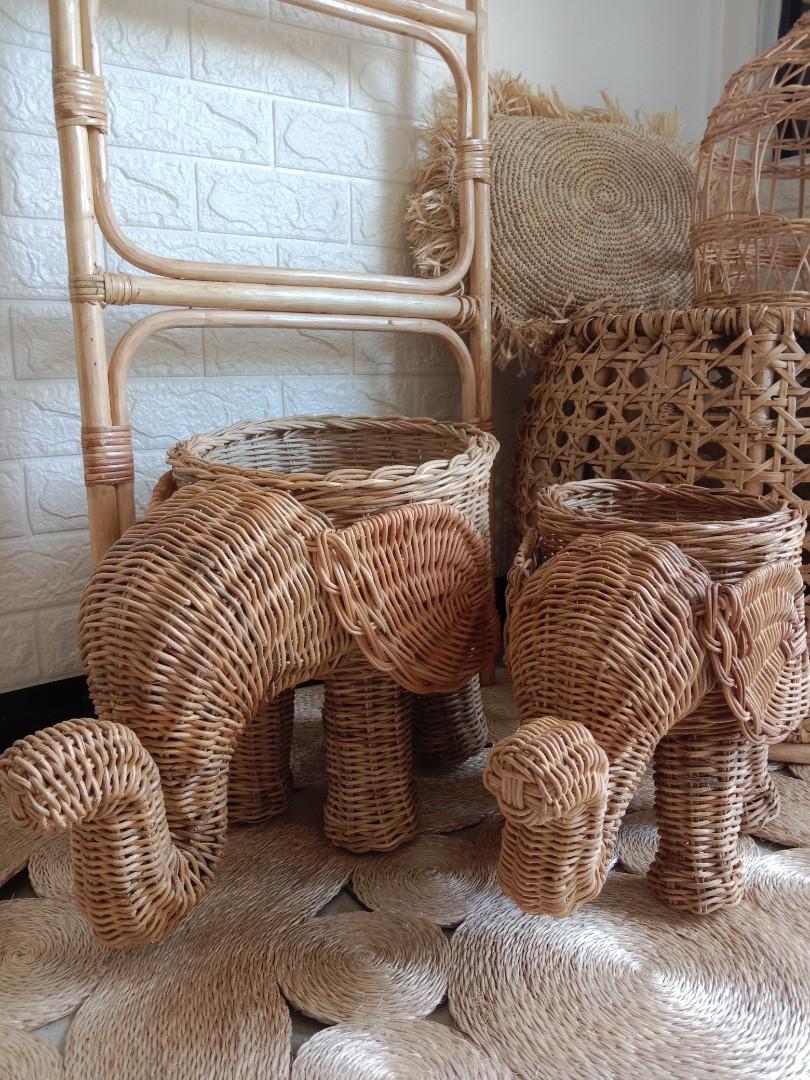In this bright and sunny room, the focal point is a pair of intricate wicker baskets shaped like elephants, with the one on the right slightly smaller than the one on the left. These unique elephant baskets are set against a white brick wall that features various patterned indentations, adding subtle texture to the background. Beneath the elephants lies a rug made of coiled wicker material, composed of numerous circular and floral shapes that conceal the floor. To the left of the elephants stands a wooden and wicker ladder-like sculpture, held together by rope coils, while larger traditional wicker baskets are positioned to the right. Additionally, a bamboo frame and a birdcage made of dried reed can be seen in the background, further enriched by the light brown and white color scheme of the room.